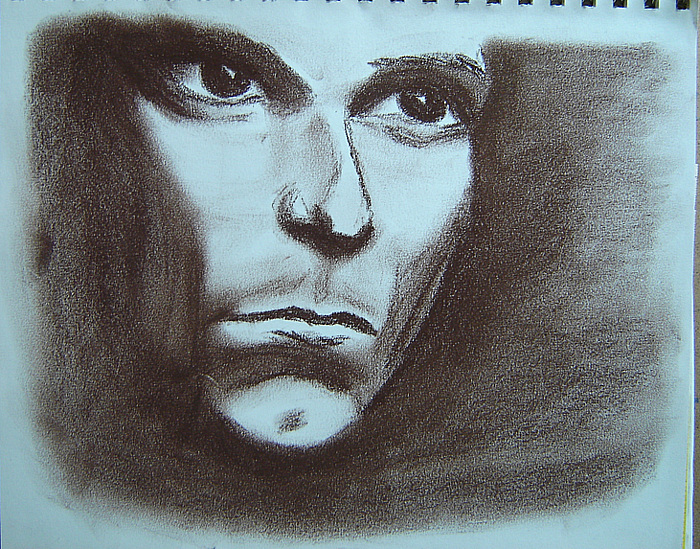The image is a sketch that appears to be captured as if someone took a photo of a drawing, looking directly down at a notepad or sketchbook. The paper in the sketch has a bluish hue, which might be due to white balance effects in the photograph, or it may actually be blue paper. The drawing itself depicts a face, with the artist employing negative space to define the lighter areas of the skin rather than drawing them outright. The dark regions are rendered with charcoal, creating smudged, textured effects. The face in the sketch is of a man looking to the right, with the use of charcoal giving depth and contrast to the image.